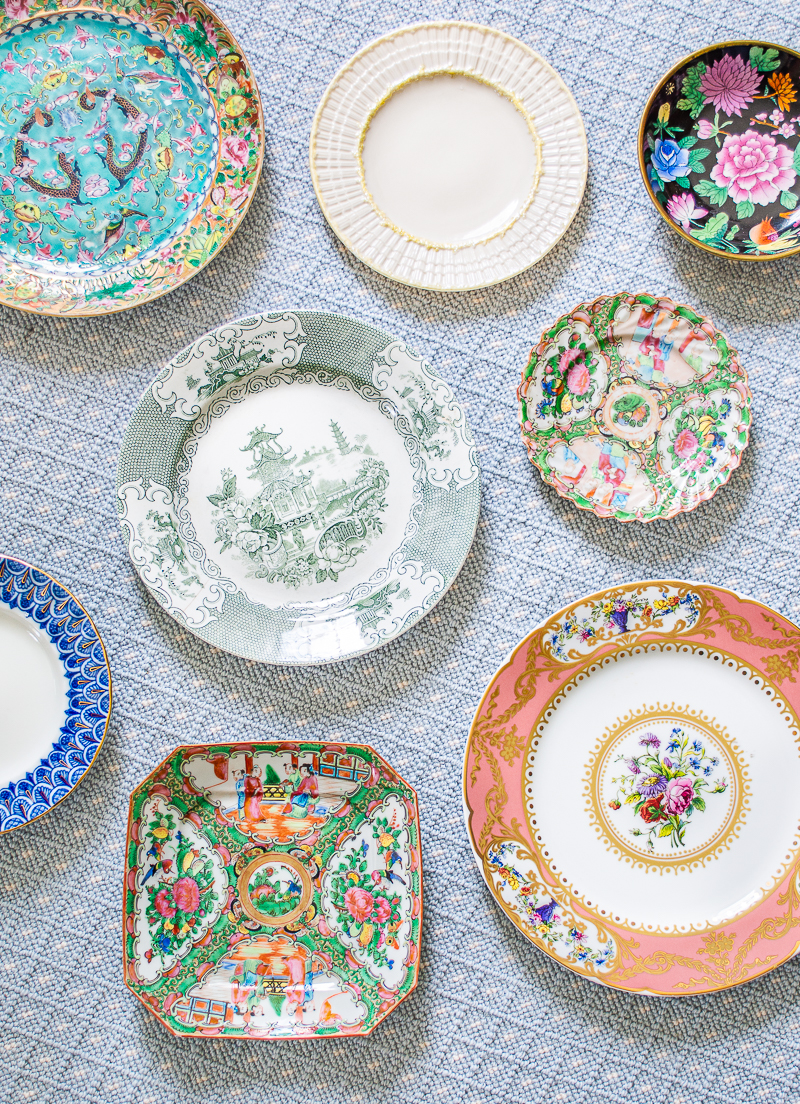The image features eight ornate antique plates, each with a unique design. Displayed in an overhead shot on a light blue grid-patterned cloth, the plates form three rows: three on the top, two in the center, and three at the bottom. The top-left plate stands out with bright blue and vivid pink colors, the middle plate is slightly smaller with cream-white and gold accents, and the top-right plate is the smallest with a black background adorned with bright flowers. The center row showcases a large plate on the left with a white base and jasper green chimoise design and a smaller plate on the right with pink, blue, and green floral patterns. The bottom row includes a plate partially cut off on the left with a bright blue edge and white center, a square plate in the middle featuring green, yellow, and pink flowers, and the largest plate on the right with a coral-peach rim, white inner circle, and pink flower center. The intricate and colorful designs, ranging from red, pink, yellow, blue to black and white, along with combinations of circular and square shapes, make this collection visually appealing and likely indicative of expensive antiques.